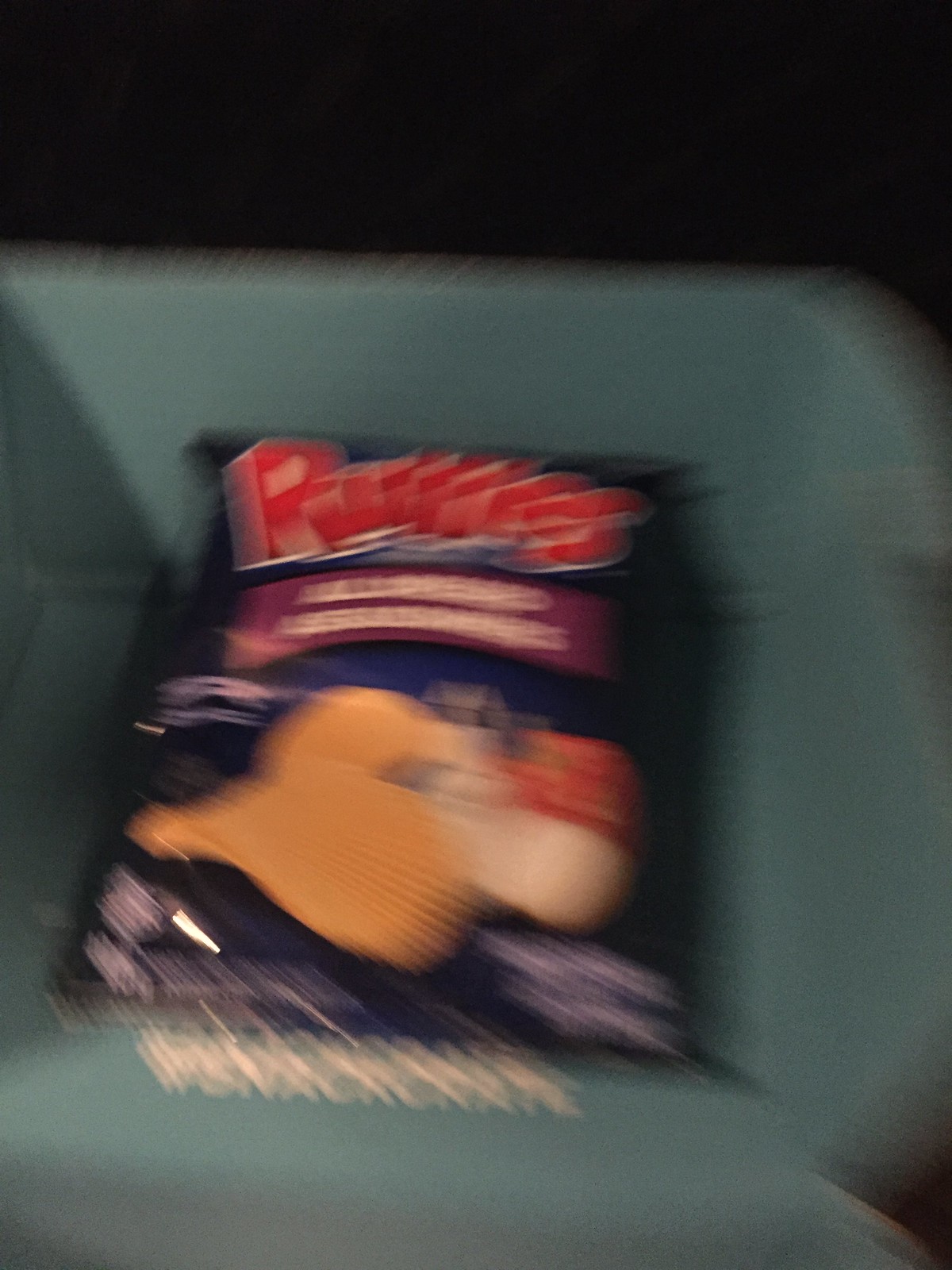This photograph features a blue bag of Ruffles chips resting on what appears to be a blue cloth chair. The image is highly blurry, making the details difficult to discern. At the center of the image, the Ruffles bag displays red lettering prominently, while beneath the Ruffles logo, there is a purple ribbon with text. Below the ribbon, one can make out the blurred shapes of potato chips and a red vegetable, possibly suggesting a flavored variety. Additionally, the bag contains areas of white text, though they are not easily readable due to the blurriness of the photograph.